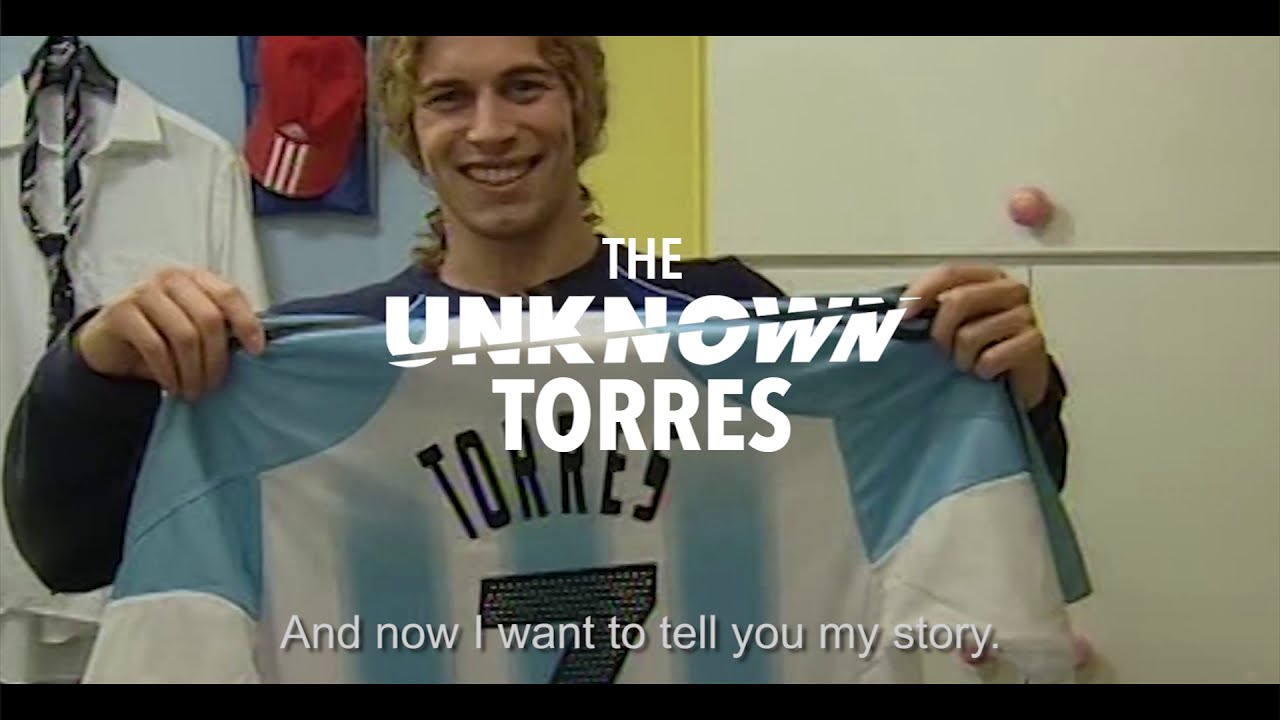The image appears to be a high-definition still from a video, likely showcasing a personal story of an athlete. It features a young white man with long blonde hair tied back in a ponytail, smiling directly at the camera. He is proudly holding up a sports jersey, which is predominantly light blue and white, with the name "Torres" (T-O-R-R-E-S) in black text and the number seven beneath it. He is dressed in a blue long-sleeved shirt. The setting seems to be a locker room or a personal room, evidenced by various items in the background: a suit with a blue tie on a hanger, a red baseball cap with white stripes, and white closets. Superimposed on the image, in the center, is white text reading "The Unknown Torres," while at the bottom, there is a caption that says, "And now I want to tell you my story." This screenshot likely serves as a promotional image for a video narrative about the athlete's life.